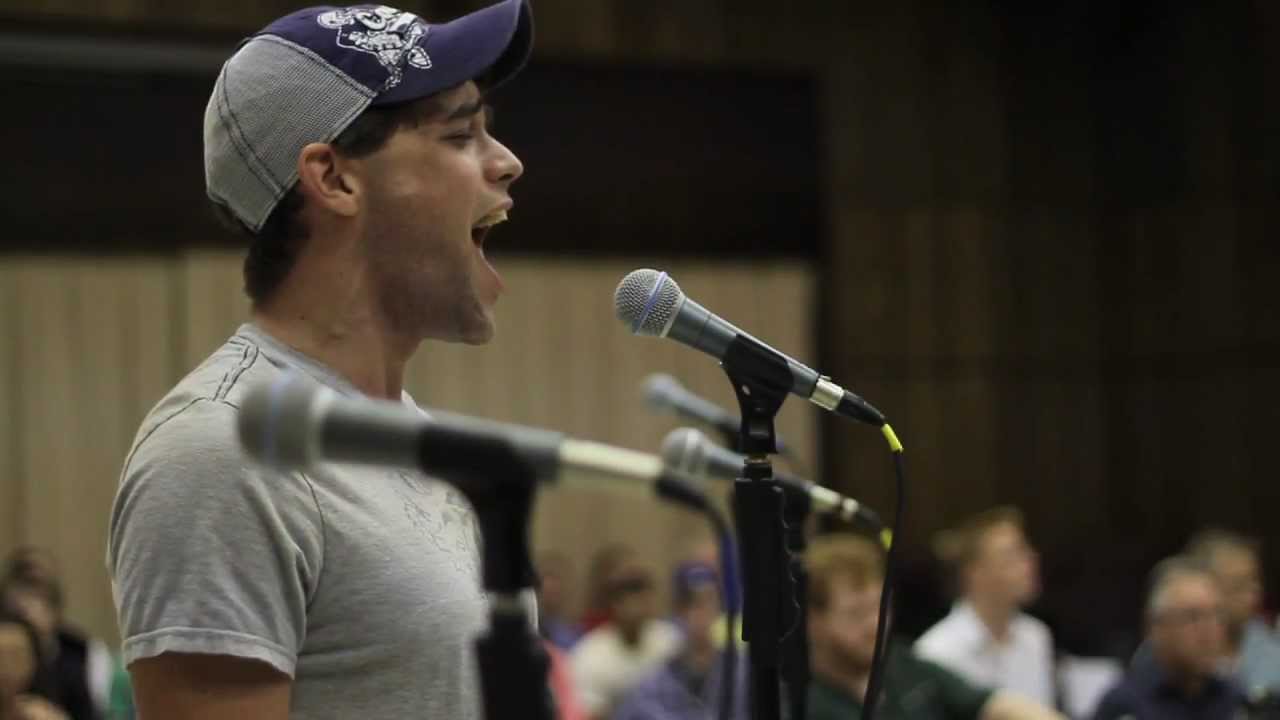In this image, a brown-skinned man, presumably Latino and with short dark hair, stands on a stage indoors, passionately singing into a silver microphone mounted on a black stand. He is positioned to the left side of the frame and wears a light gray t-shirt and a gray and purple baseball cap adorned with some artwork or logo on the front. His eyes are closed as he sings, suggesting deep emotion. Surrounding the main microphone are at least three additional silver microphones, each connected with black cords. In the background, a group of blurry, attentive people sits among a mix of white and brown walls, appearing to be in an auditorium filled with rows of chairs. A curtain also seems to be present behind him. The setting is well-defined by the various elements, indicating a live indoor performance.